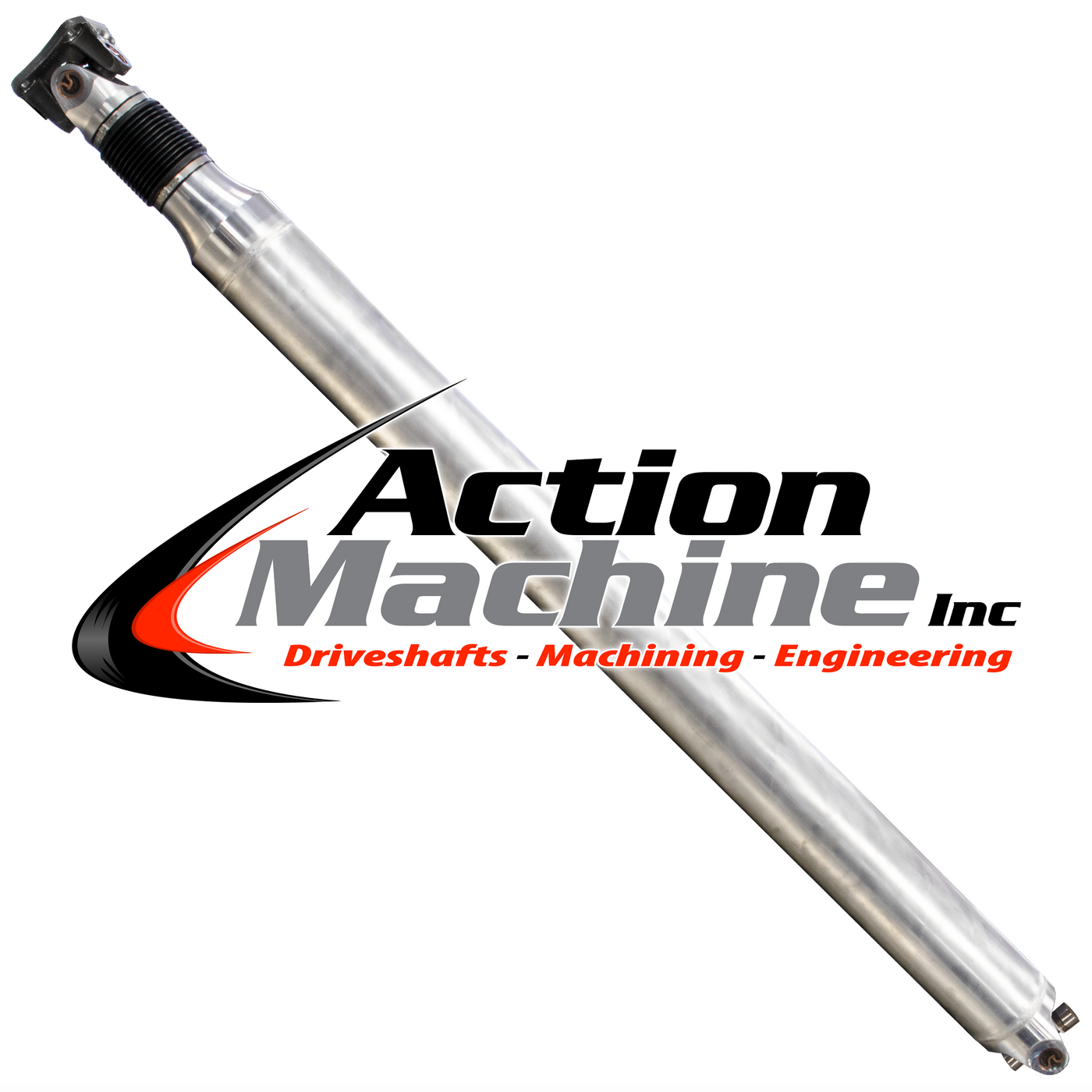The image depicts a drive shaft, an automotive part, presented prominently in the photograph. The drive shaft is placed diagonally, extending from the top left corner to the bottom right corner of the frame. This cylindrical, metallic rod has a glossy finish, hinting that it might be made of aluminum or steel. The main body of the shaft is silver-grey in color, and it becomes slightly thinner towards the top left end. At this thinner end, there is a black band, followed by a small cylindrical black piece with a screw attachment. 

Centrally positioned on the image is text in black and grey, reading "Action Machine Inc." The text includes a curving logo with black and red elements. Below this, in smaller red letters, the text reads "Drive Shafts, Machining and Engineering." Overall, the composition highlights the sleek and precise design of the drive shaft while simultaneously emphasizing the branding and product description.